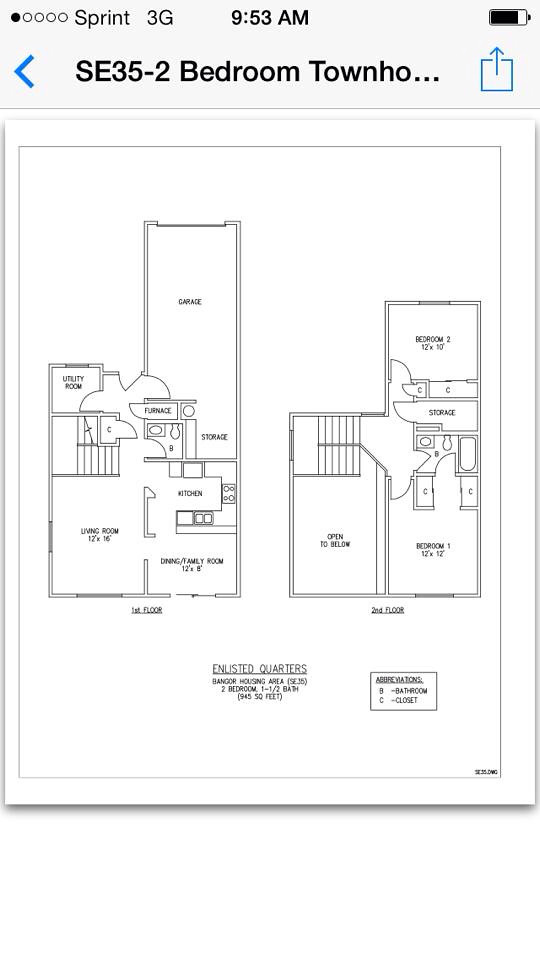This is a detailed screen capture from a mobile phone displaying a floor plan. In the top right corner, the screen reads "Sprint 3G," indicating the network status. Just below that, it shows the time as "9:53 AM" and the battery icon, which is approximately 80-85% charged. Below the battery icon, the text reads "SE35-2 Bedroom Town", followed by "HO..." with three dots suggesting truncated text. On the left side of the screen is a blue arrow pointing to the left, and on the far right, there is a blue square with an arrow emerging from it pointing upwards.

At the bottom of the screen is a white square with a black border inside, which contains the detailed floor plan. The plan includes labels such as "garage," "utility room," and "living room" on the first floor, alongside "dining," "family room," and a note labeling this section as the "first floor." The second floor shows labels for "bedroom 1," "bedroom 2," "storage," and the label "open" for an unspecified area. At the very bottom, the text "enlisted quarters" is visible, but the writing below it is too faint to decipher, as is much of the writing within the floor plan itself. There is also a smaller, hard-to-read square next to the main floor plan with indecipherable text.